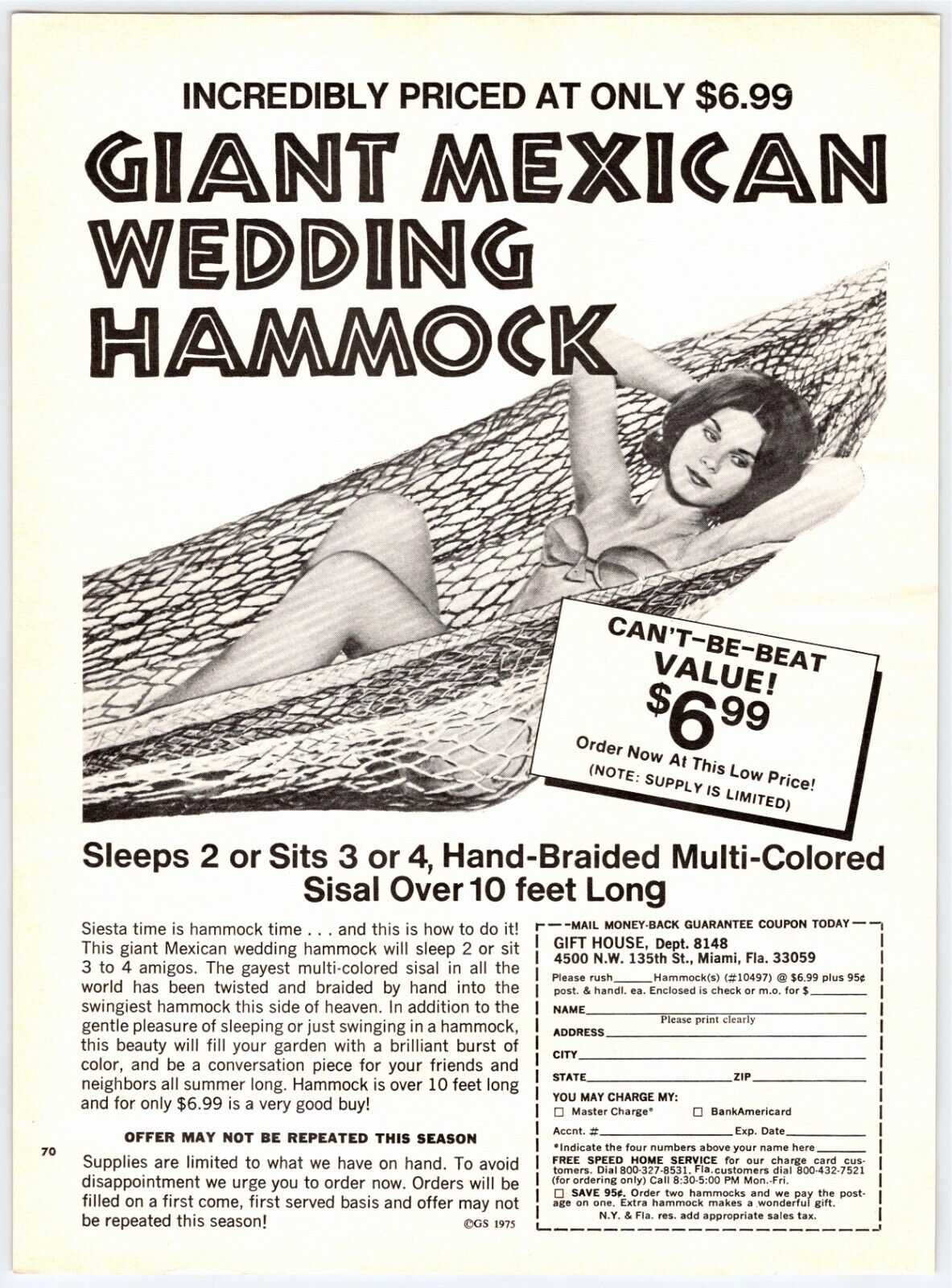This vintage advertisement features a yellowing border, indicating its age, and is set against a white background. The header reads, "Incredibly priced at only $6.99," emphasizing the affordability of the product. Below the header in bold, dark black font, the ad proclaims, "Giant Mexican Wedding Hammock."

Centrally placed, the image showcases a woman dressed in a string bikini, reminiscent of 1960s fashion, lounging in the hammock with her hands behind her head. The ad reiterates the unbeatable value with the text, "Can't beat this value, $6.99." 

A coupon is provided in the lower section, reinforcing the magazine-style presentation, inviting readers to mail in their order. The company, "Gift House," based in Miami, Florida, details the product's features: it can comfortably sleep two people or sit three to four, is hand-braided, multicolored, and spans over 10 feet in length. 

The overall aesthetic and pricing point solidify the advertisement's dated charm.